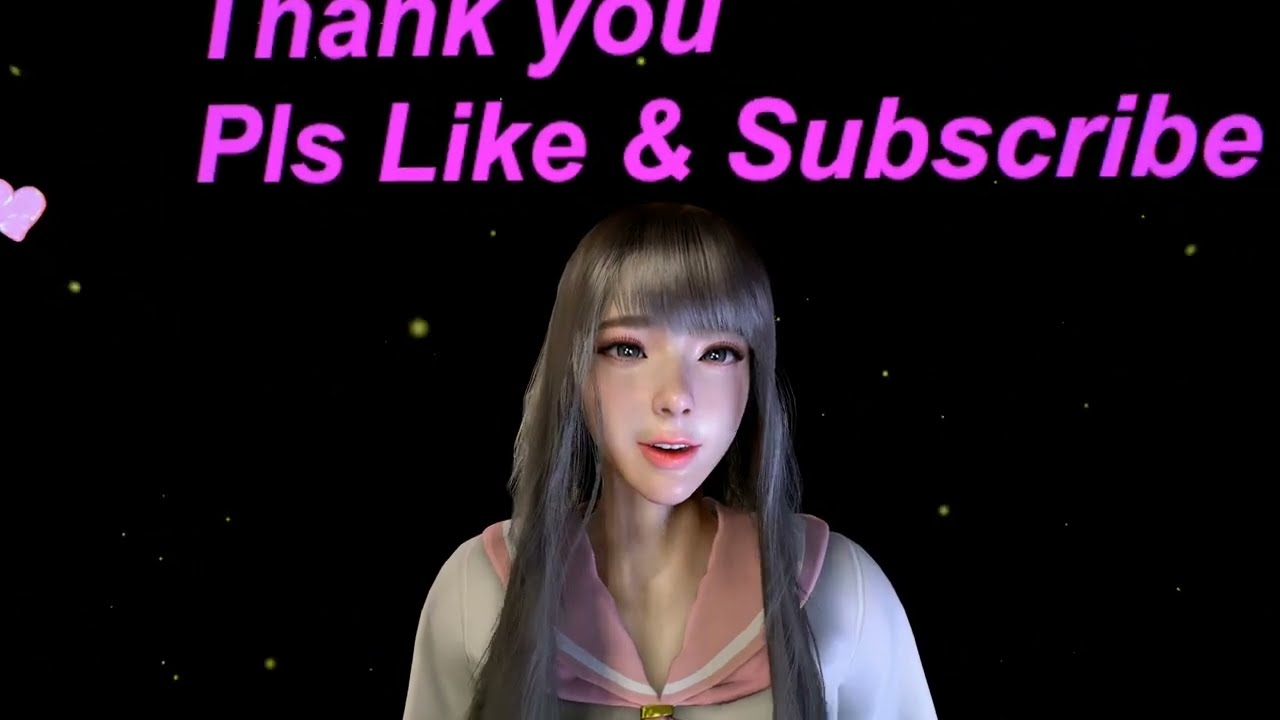In this digitally created image, a central animated woman stands out against a predominantly black background speckled with yellow dots resembling stars, suggesting a night setting. The woman has long, flowing silver hair with bangs that extend past her eyebrows, and her gray eyes highlighted by mascara and eye makeup are clearly visible. She has a slight smile on her face, revealing the top of her teeth as if she might be speaking. Dressed in a pink and gray blouse with a flesh-tone collar and what appears to be a gold clasp at the bottom, she exudes a serene presence. Positioned just above her head in pink text, it reads, "Thank you PLS like and subscribe," with an incomplete heart icon nearby on the upper left side of the image. The overall aesthetic suggests this is an animated scene likely intended for a YouTube channel or similar digital platform.